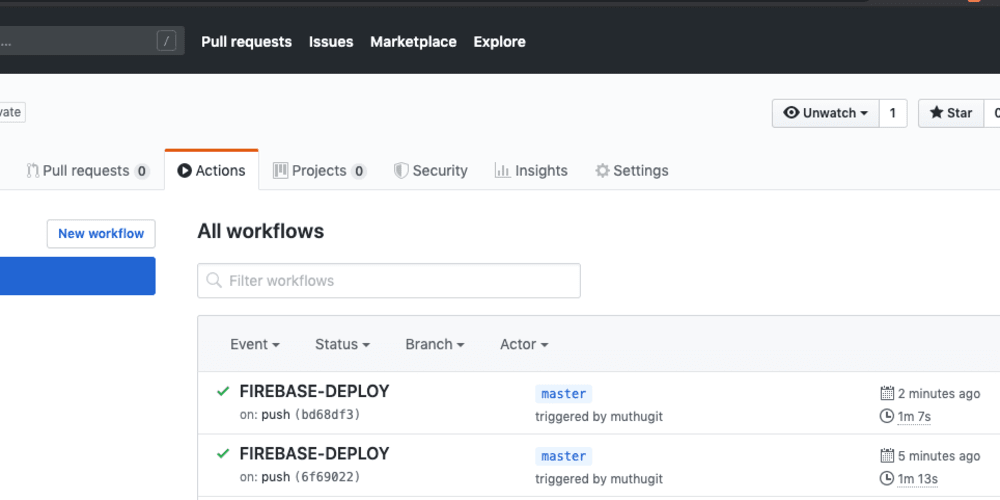This is a screenshot of an application interface, displaying several navigation and menu options. At the top, there is a horizontal black bar containing four menu items: "Pull requests," "Issues," "Marketplace," and "Explore." Below this, on a white background, there is a secondary menu featuring five tabs: "Actions," "Projects," "Security," "Insights," and "Settings." The "Actions" tab is active and selected. Within the "Actions" section, it shows a subheading labeled "All workflows," accompanied by an empty dialog box intended for filtering workflows by specific terms. Beneath this filter box, two workflows named "Firebase Deploy" are listed.